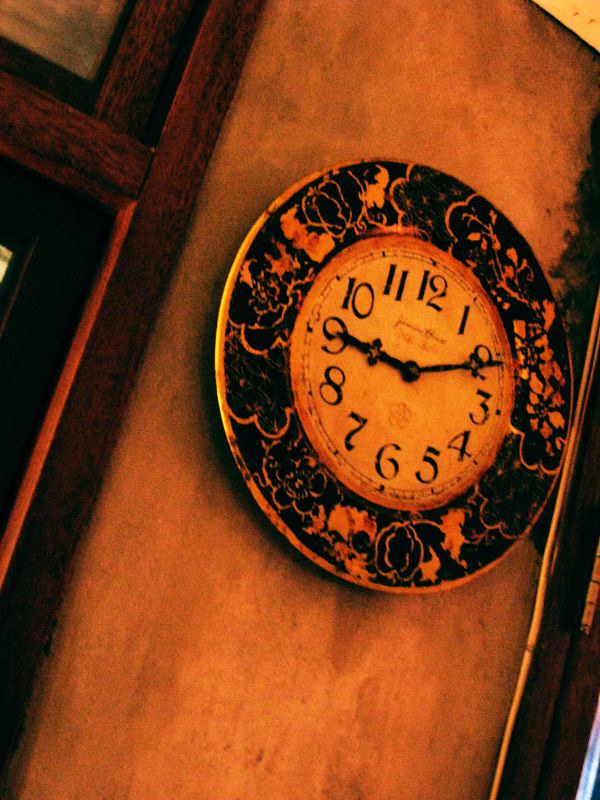The image is vertically taller than it is wide, featuring a warm, orange hue that suggests the lighting effect of a late evening sunset enveloping both the background and foreground. Dominating the center is an intricate analog clock, positioned diagonally such that the 12 is more at 12:30. The clock rests against an off-white, stone-like wall. Flanking the clock, there appears to be dark brown wooden elements, possibly the edges of doorways or window sills. The clock itself is decorated with an ornate floral pattern comprising black and orange-tinted flowers due to the sunset glow. The clock's face is about four inches in diameter, and the hands are set to 9:10. The entire scene gives an impression of serene twilight, enhancing the overall ambiance with a softly diffused golden light.